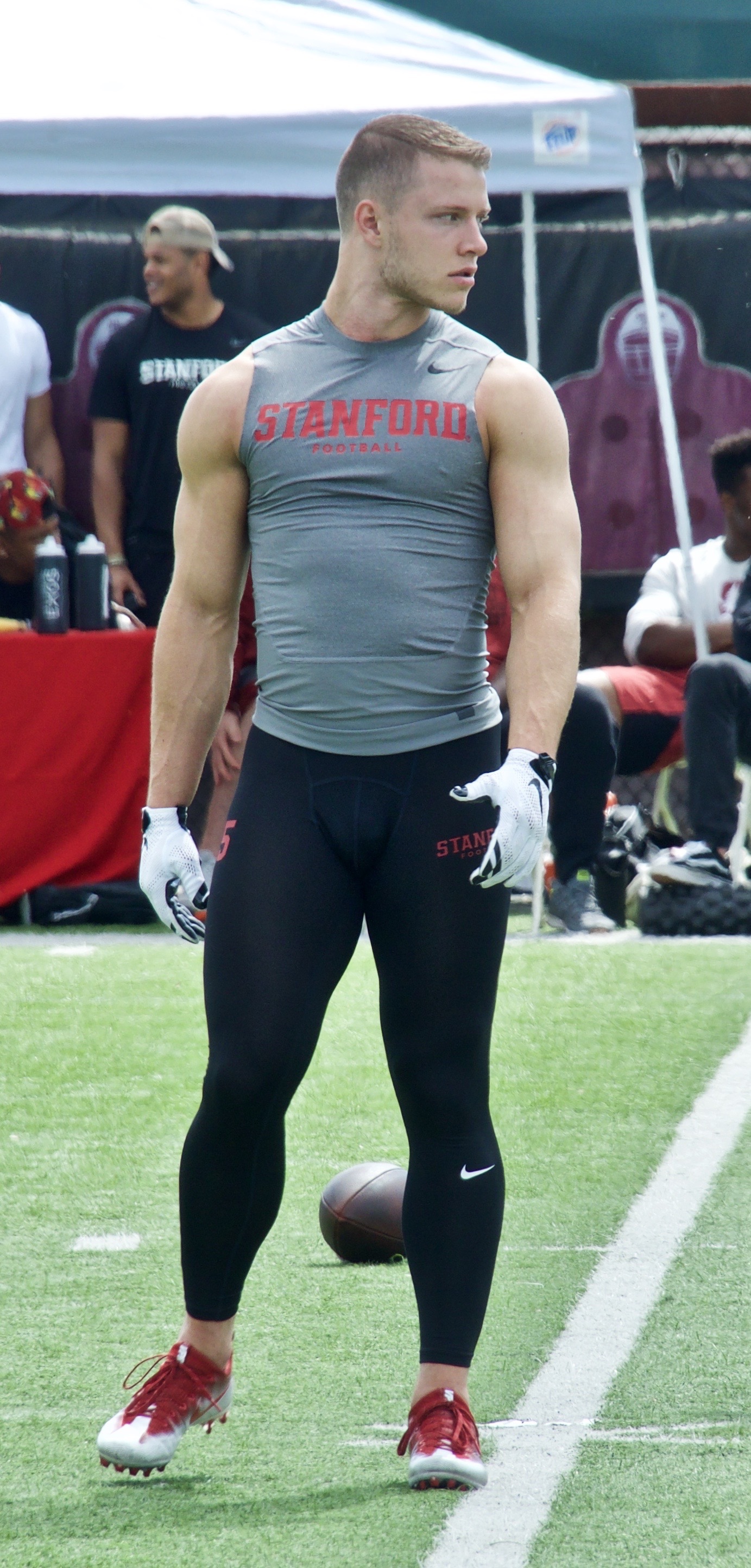In this image from what appears to be a football practice or pregame warm-up, a very fit young man in his 20s is prominently featured. He is standing on the green football field near a white stripe marker. The man is dressed in a tight, gray, sleeveless shirt emblazoned with "Stanford Football" in bold red letters on his chest, and he wears tight black spandex pants with a red "Stanford" logo on his upper right thigh. His outfit is completed with white gloves that have black accents and red and white cleats. The player’s body is facing the camera while his gaze is directed to his left, showcasing his short, light brown hair. A football is visible on the grass near his calves. In the background, there are other people, some standing and some sitting, as well as a fence and a pop-up tent with a red table and water bottles, adding to the lively atmosphere of the scene. Various football equipment can also be seen scattered around.